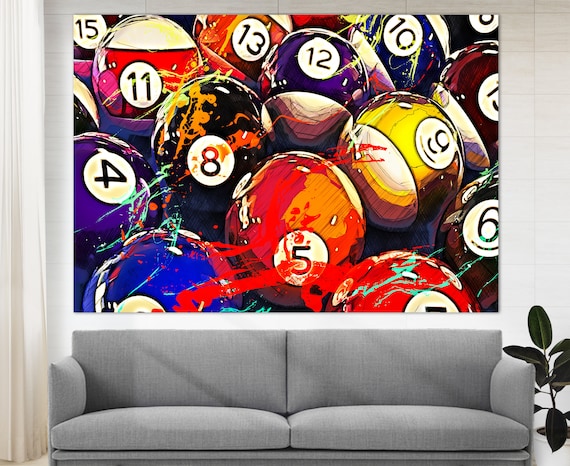This image features a gray loveseat with thin cushions and armrests, situated against a plank wall. To the right of the couch, a white ceramic planter holds a thriving ficus with large, dark green leaves. On the left side, a long white curtain cascades down, presumably covering a window. Above the couch, a large painting dominates the wall, depicting pool balls in a somewhat abstract, cartoony style. The balls are realistically colored and numbered, but splashes of paint add a whimsical touch, making the artwork vibrant and colorful. The balls feature hues of yellow, orange, black, purple, blue, and brown, with each ball displaying white stripes and numbers. The image is detailed, capturing a cozy and artistic domestic scene.